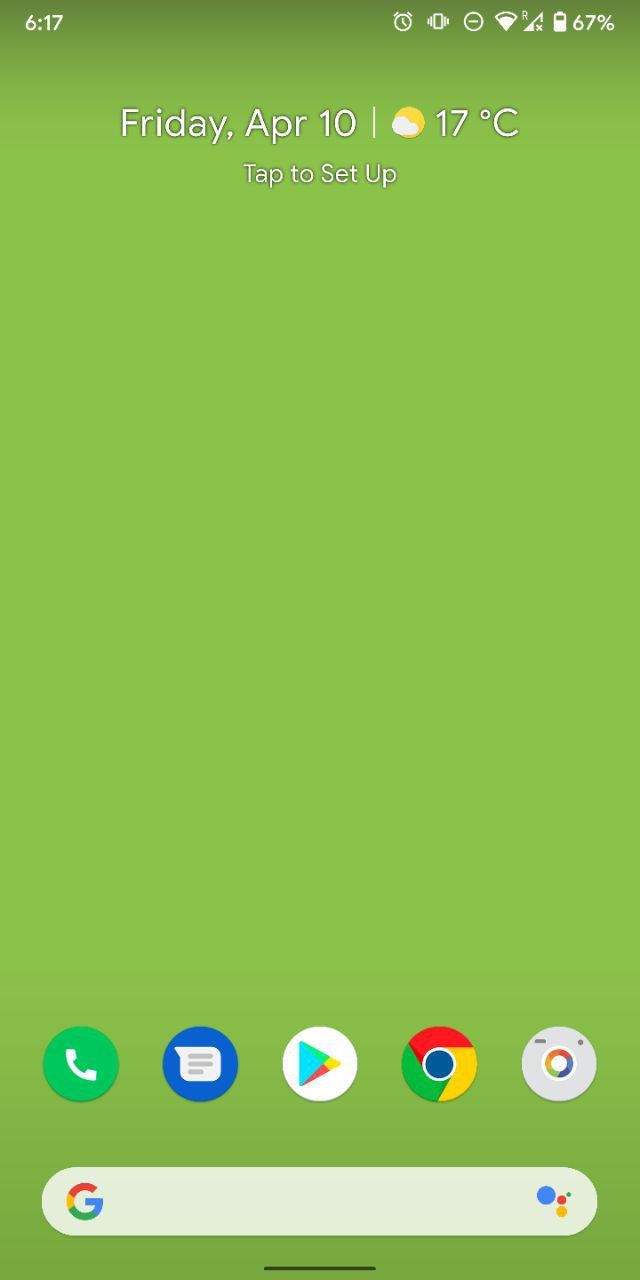This detailed description captures the elements found on an Android home screen with precision and clarity. Here is the information presented in a well-structured and descriptive caption:

---

The image depicts an Android home screen. Situated at the top left corner is a timestamp reading "6:17". Adjacent to the timestamp is an alarm clock icon. To the right of the alarm, a vibration mode indicator is visible, signified by a rectangular symbol with emanating lines. Next, a white-outlined circle containing a dash is displayed, followed by a Wi-Fi signal icon. Beside the Wi-Fi symbol is a service signal icon bearing an "X" at the bottom, which suggests that the mobile service might be turned off or restricted, indicated by an "R".

Moving further to the right, a battery icon reveals a 67% charge in white text. Below this top row, additional white text displays the date as "Friday, April 10th," separated by a white divider. Directly under the date, a weather widget shows an image of a sun peeking from behind a cloud, along with the temperature "17°C". It also includes a prompt "Tap to set up", and the text appears to be accented with a black border or shadow. 

The backdrop of the home screen is a soothing light green color. At the bottom of the screen, a Google search bar is present, featuring the traditional Google logo on the left and a speech assistant icon on the right. Above this search bar are five shortcut icons for calls, messages, the Play Store, Chrome, and an unidentified app resembling a photos icon. The overall image appears slightly stretched, making the circular icons look broader than usual.

---

This caption methodically describes the home screen's components, providing clear context and visual details.